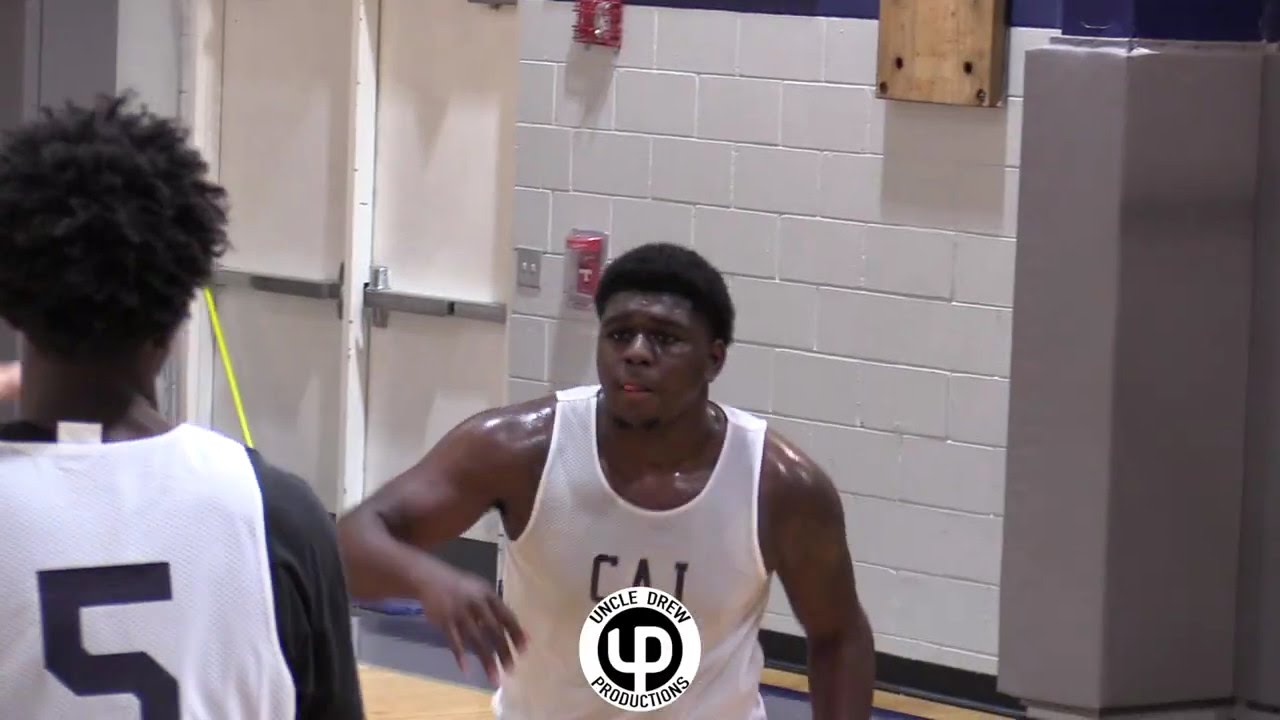In this very wide rectangular photograph, we are in what appears to be a gymnasium, possibly a high school gym, where people are playing basketball. Dominating the background is a large, gray, horizontally-bricked wall that starts at the bottom right corner and stretches diagonally upwards. Near the middle of the image, set against this wall, there's a red fire alarm adjacent to a white light switch. To the left of the switch is an off-white double door equipped with silver horizontal push handles, and further left stands a white pillar.

Central to the photograph is a black man, visible from the torso up, who is sweating profusely. His hair is slightly puffy and he is wearing a white basketball jersey. He looks focused and is gazing towards the left side of the image. On the left side of the frame is the backside of another black man with frizzy hair, wearing a black jersey with the number five on it. He is also wearing a black t-shirt underneath his jersey. 

At the bottom center of the image is a logo that reads "Uncle Drew Productions," adding a unique textual element to the scene. The overall color palette includes shades of white, black, gray, light brown, red, yellow, and tan, reinforcing the setting's gymnasium ambiance.